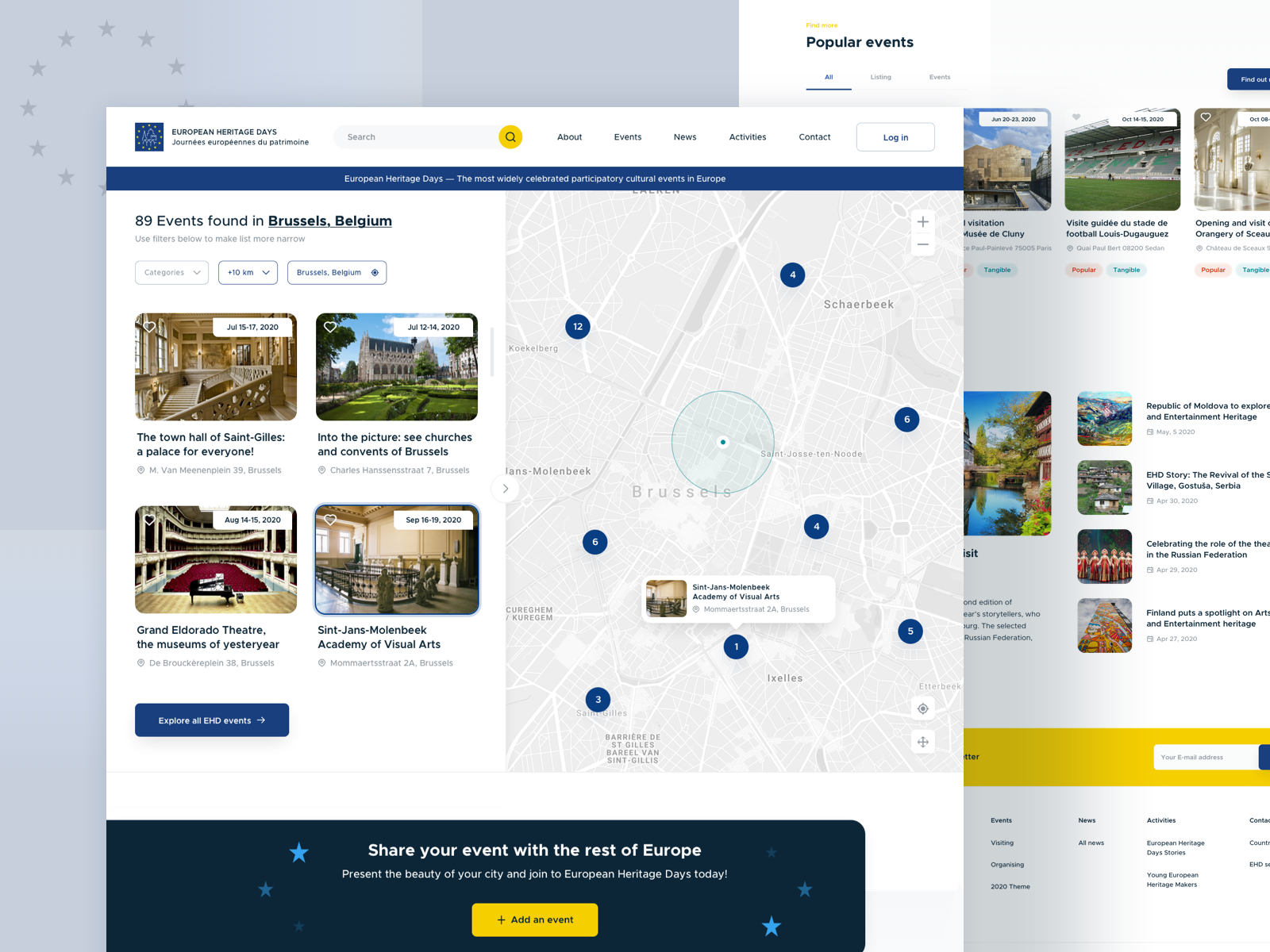The image is divided into two halves with distinct backgrounds: the right half is white, while the left half is a light blue hue. Central in the foreground is a webpage highlighting "European Heritage Days." The top left of the page showcases the text: "European Heritage Days, Jeunesse Européenne du Pachamonnet, Némesis-Echeba." 

In the upper right corner, navigation tabs include About, Event, News, Activities, Contacts, and Login. Beneath these tabs, against a blue backdrop, bold white text reads: “European Heritage Days, the most widely celebrated participatory cultural event in Europe.”

On the left side of the page, a filter section shows "89 events found in Brussels, Belgium." Users are prompted to use filters like "Category" and "10-kilometer radius" to narrow the list.

Highlighted events include:

1. "The Town Hall of Saint-Gilles: A Palace for Everyone" - showcasing a palace with light brown colors.
2. "Into the Picture: See Churches, Halls, and Convents in Brussels" - featuring an image of green grass and buildings.
3. "Grand Eldorado Theatre: The Museum of the Easter Year" - presenting a museum interior with red seats and a brown piano.
4. "Saint-Jean’s: More Than Big, Academy of Visual Arts."

A blue button at the bottom left says "Explore all EHT events." An invitation text below reads, “Share your event with the rest of Europe, present the beauty of your city and join European Heritage Days today.” Below this is a yellow button labeled "Add an Event."

To the right, a map of Brussels displays blue numbered markers (4, 1, 3, 4, 4, 5, 6, 6, 12). In the background, faint images of locations are visible, though partially obscured.